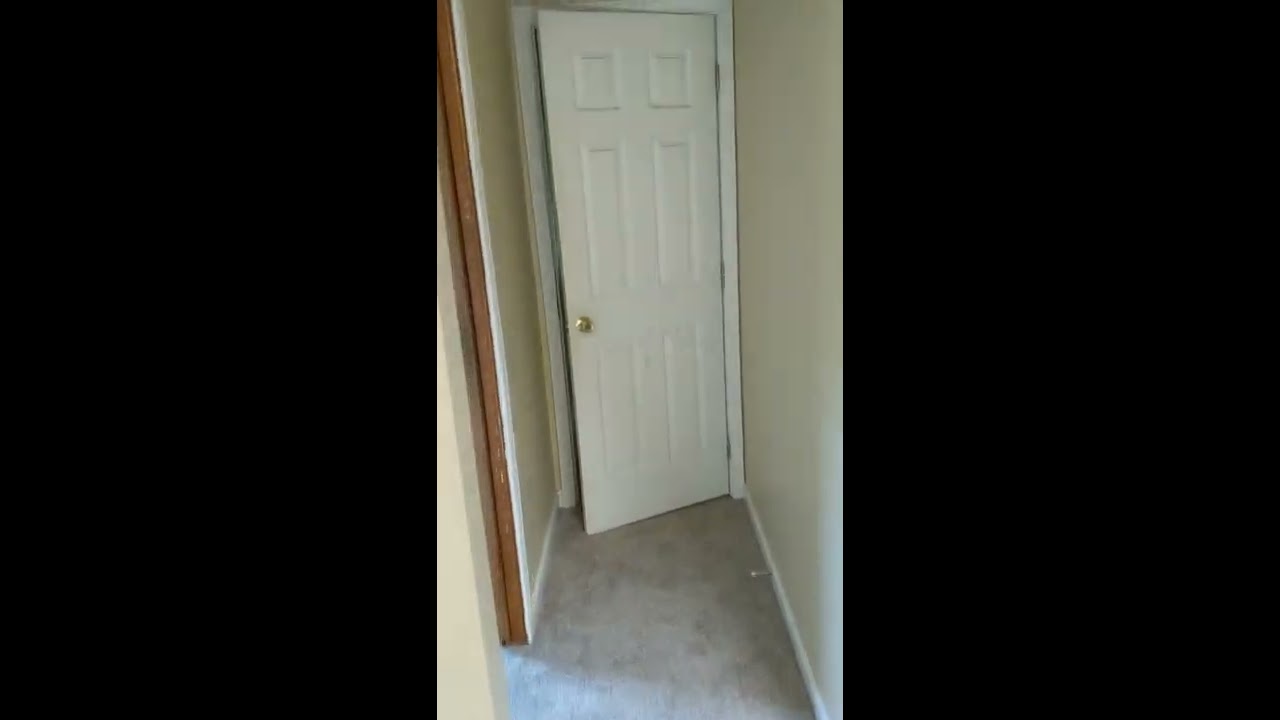This detailed photograph captures a narrow hallway within a home or apartment, characterized by off-white walls and pure white trim and baseboards. The floor is covered in gray carpeting. A partially open white door stands directly at the center, featuring a gold doorknob and ornate rectangular indents. Indistinct yet visible, there’s a door stop situated near the base of the right wall, which is designed to protect the wall from damage when the door is opened. An open doorway to the left reveals natural wood tones on its interior, though the room beyond is not visible. Subtle light filters through this left doorway, illuminating a portion of the carpet. The image itself is bordered by thick black margins on the left and right sides, giving an almost framed appearance, and lacks any textual elements. Overall, the setting conveys the impression of a new or sparsely decorated home space, potentially part of a video capturing more of the surrounding environment.